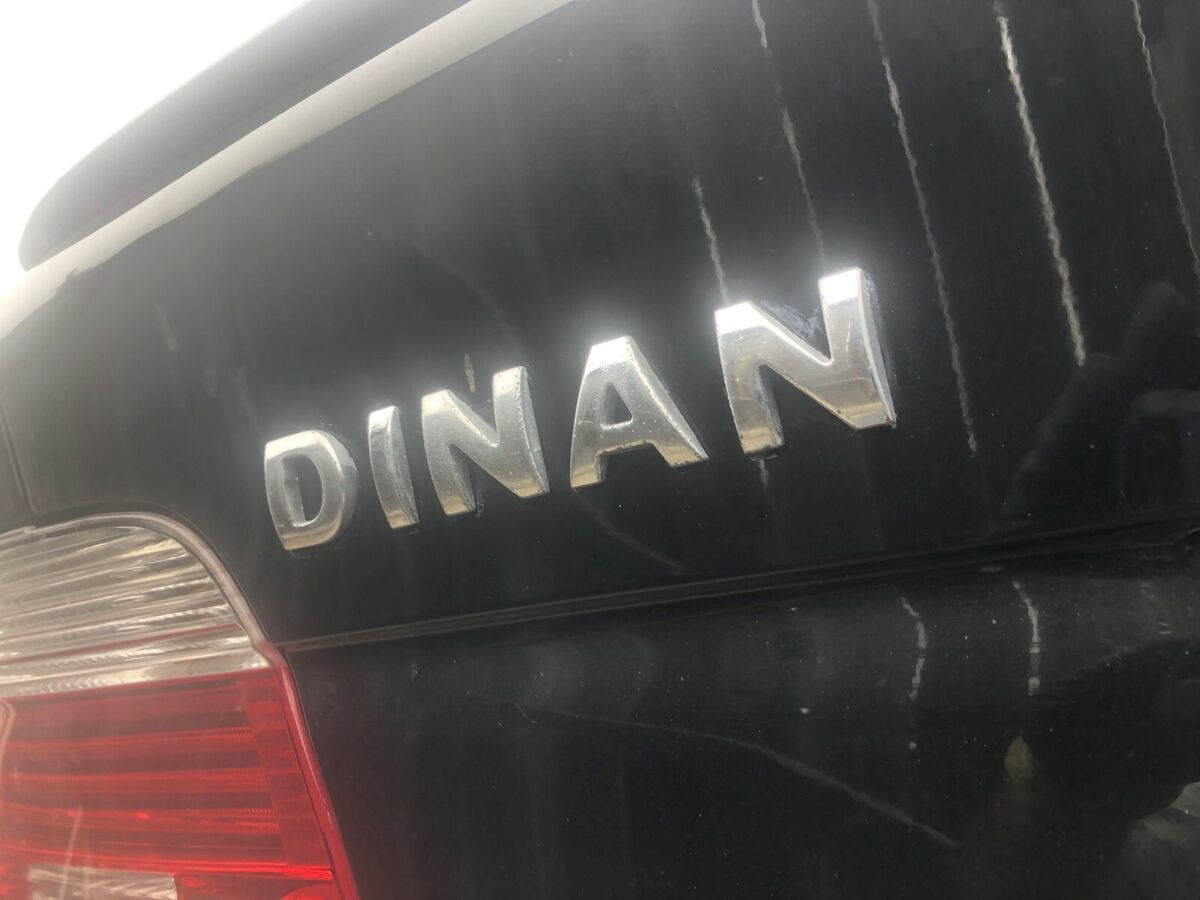This close-up photograph of a black sedan vehicle was taken on an overcast day, with a clear gray sky in the background. The picture is tightly focused on a section of the car, revealing a variety of details. In the bottom left-hand corner, part of the taillight is visible, which has a white upper part and a red lower part, both made of plastic. Adjacent to the taillight, the word "Dinan" is displayed in silver reflective letters, positioned on what might be the rear bumper or a grill-like structure with white horizontal stripes. The upper left-hand corner of the frame captures a bright white area, and the overall image showcases reflections off the vehicle’s glossy black paint. There is also an indistinct feature at the top of the image that might be a spoiler.